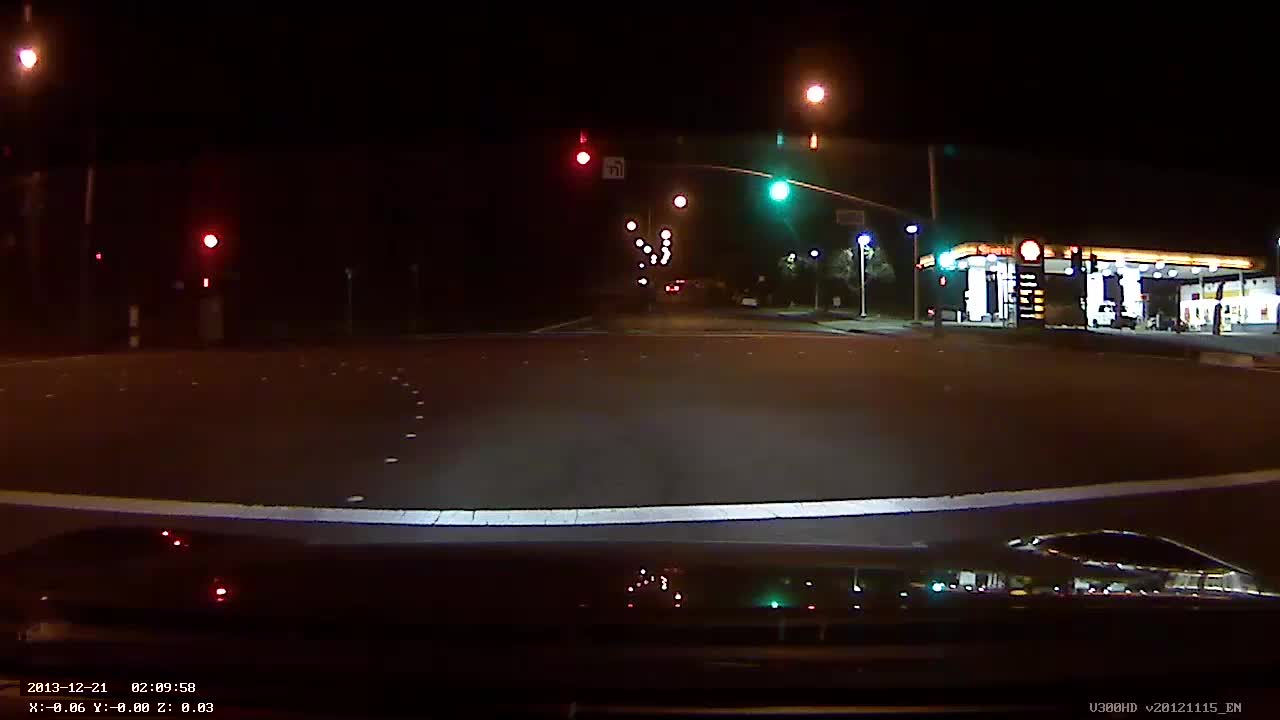In this nighttime dash cam image, we are looking through the windshield of a car, apparently waiting at a red light. The sky is pitch black, enhancing the brilliance of streetlights and the illuminated elements in the scene. Directly in front of the car, the roadway extends forward with two lanes visible on either side. The top of the car, shiny from the lights, suggests it's slick with reflection. 

To the right side of the image, a well-lit Shell gas station with a convenience store and multiple bays stands prominent. The station's logo—a distinctive yellow shell—is clearly visible atop the sign. Nearby, a gas price sign is faintly discernible but too distant for the numbers to be read. Several cars can be seen at the gas station, adding to the scene's nocturnal ambiance.

Above the roadway, a traffic light displays a red signal for the lane the car occupies, while a green light on the right is possibly for a different lane. Additional street lights cast halos in the background, indicating it's a well-illuminated area. Another red traffic light can be spotted in the left side of the frame. 

The bottom left corner of the image shows a timestamp of 2023-12-21 and the time 02:09:58 AM, along with some numerical coordinates and a product code that's difficult to decipher due to its small size. The bottom right corner also contains some small, unreadable white font.